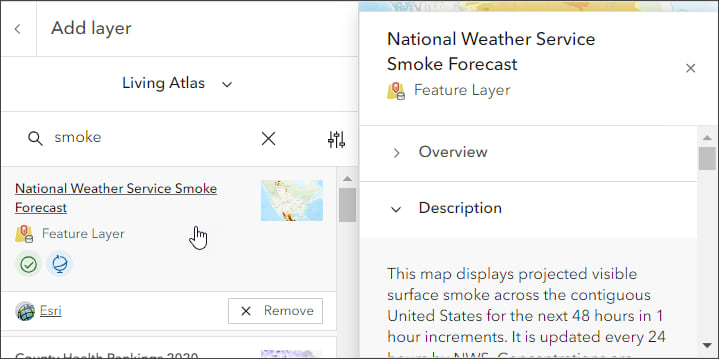A landscape-oriented screenshot from an application interface, likely related to coding or data visualization, featuring a thin black border. The rectangular image, approximately twice as long as it is tall, is split into two main sections.

On the left side, a gray panel features a navigation button in the top-left corner with a left arrow and the label "Add Layer" in black. Below this, a divided area titled "Living Atlas" includes a drop-down box. Directly underneath is a white search bar with a magnifying glass icon and the search term "Smoke," accompanied by an X and a Filters tab. Further down, a grayed-out section titled "National Weather Service Smoke Forecast" includes an underlined title and a U.S. map icon, followed by an outlined grid image labeled "ESRI" and a Remove button.

To the right, a white panel displays the title "National Weather Service Smoke Forecast Feature Layer." This panel is divided into an "Overview" section and a "Description" section, the latter being expandable with a downward caret. The description is set against a gray background with faint gray text, and includes a toggle arrow on the right for reading more details.